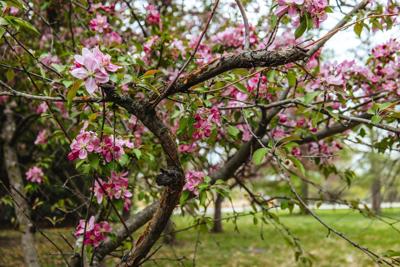This image captures a close-up view of a scraggly tree in full bloom during spring. The foreground is dominated by thick brown branches intertwined with vibrant vines, displaying an array of light pink to dark pink flowers. Interspersed among the branches are striking clusters of flowers, some almost white, highlighting the blooming season. The background reveals a blurry mix of green grass and a series of thin trees, with patches of sunlight filtering through, suggesting a bright and sunny day. Some green leaves are visible underneath the blooms, further emphasizing the season's vibrancy. The clear, white sky and a hint of a road in the background add depth to the natural scene, culminating in a beautifully detailed showcase of springtime's splendor.